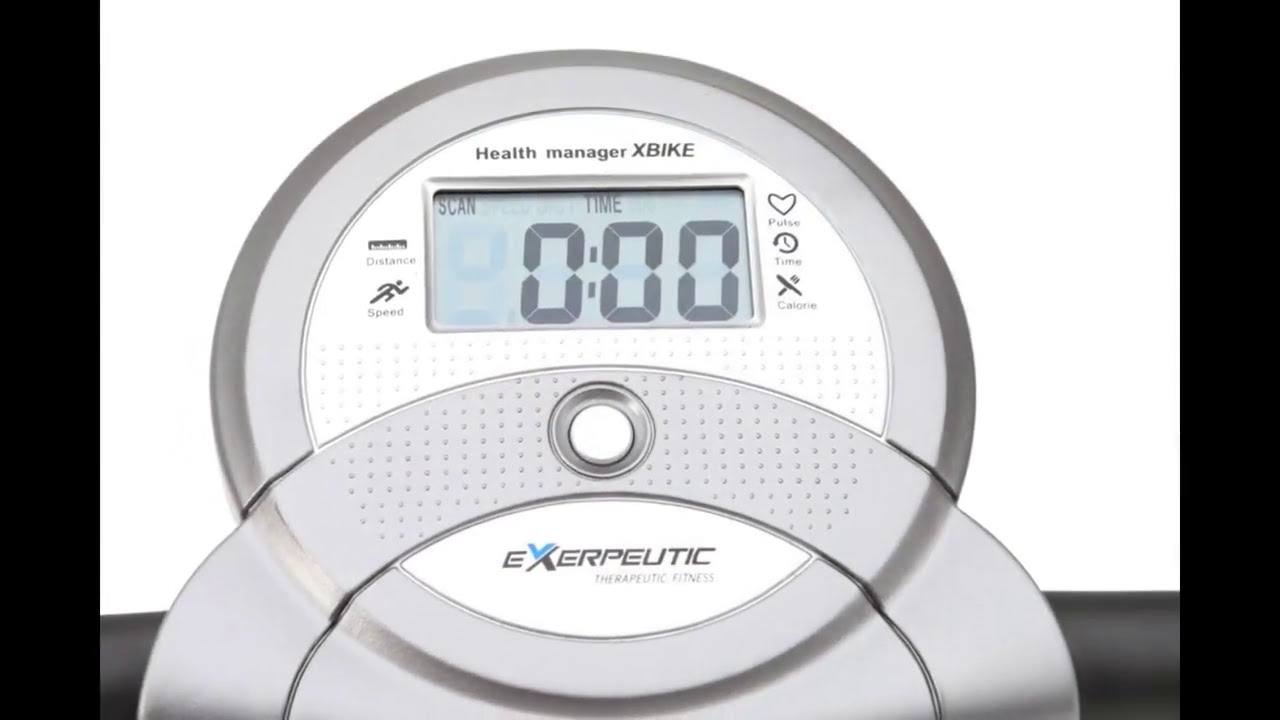This image focuses on the control panel of an exercise bike, prominently featuring a multi-layered, circular interface. The interface consists of an inner white disc bordered by a gray ring trimmed in black, all set within a larger overlapping gray disc. Centered at the top, gray text reads "Health Manager X-Bike." Below this text is a rectangular digital display showing "000," above which is the word "Time." The display resembles an old alarm clock, with additional indicators around it. On the left side, the words "Scan," "Distance," and "Speed" are visible, accompanied by a running man icon. On the right, the phrases "Pulse," denoted with a heart icon, and "Calories," represented by a fork and knife icon, are present. Beneath the main display, a prominent white push button sits centrally. The lower part of the gray disc features the branding "Exerpeutic Therapeutic Fitness," with the 'X' highlighted in blue and gray. The entire setup of this exercise bike screen represents a detailed and functional interface for monitoring various fitness metrics.